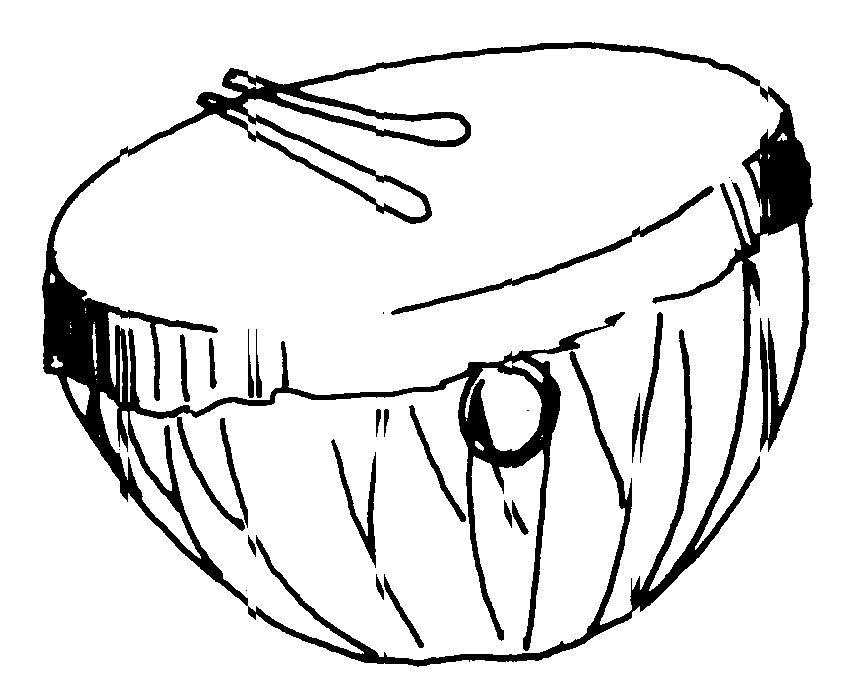The image features a hand-drawn sketch of a large timpani drum, depicted in stark black and white. The drum appears to float in a white void, emphasizing its stark, minimalist representation. The central figure is a bowl-shaped drum with a taut, circular top. Two cylindrical drumsticks with bulbous ends rest atop this surface, oriented diagonally. The drum's sides are accented with rings and various diagonal black lines, adding texture and dimension. The sketch exhibits some misalignment, likely due to the method or quality of drawing, creating an impression of charming imperfection. Shadows and textured lines provide depth, despite the simple two-tone palette. The overall style suggests an artistic rendering, possibly done by hand or digitally on an iPad. The drum is positioned slightly leaning to the left, adding a dynamic element to the composition.